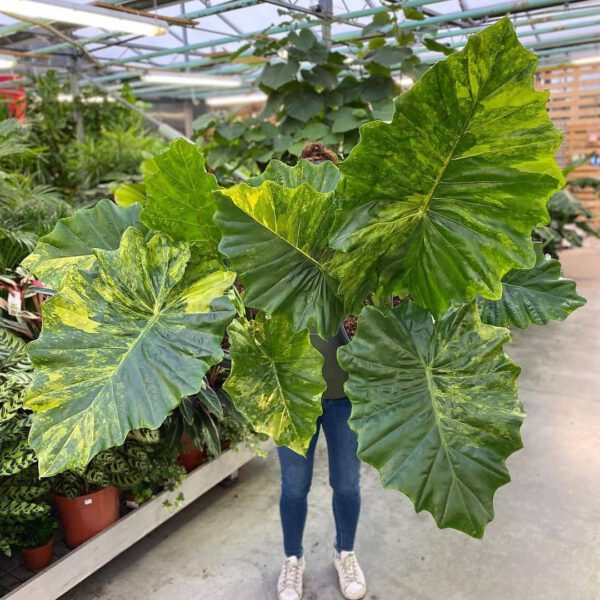In this square-cropped mobile photograph, a person stands in a well-lit greenhouse holding a large potted plant with seven to eight enormous leaves. These dark green leaves, accented with lime green and yellow spots, are so vast that they almost entirely obscure the individual, revealing only the top of their hair—likely brown and pulled up into a bun—along with their blue jeans and white shoes. The greenhouse environment features a concrete floor, a wood grate in the top right corner, and a hanging fluorescent light in the top left. Surrounding the central figure are various potted plants, with terracotta-colored pots and a background filled with lush green leaves. The greenhouse itself is characterized by its metal structure and pallets, adding to the industrial yet vibrant atmosphere of the scene.